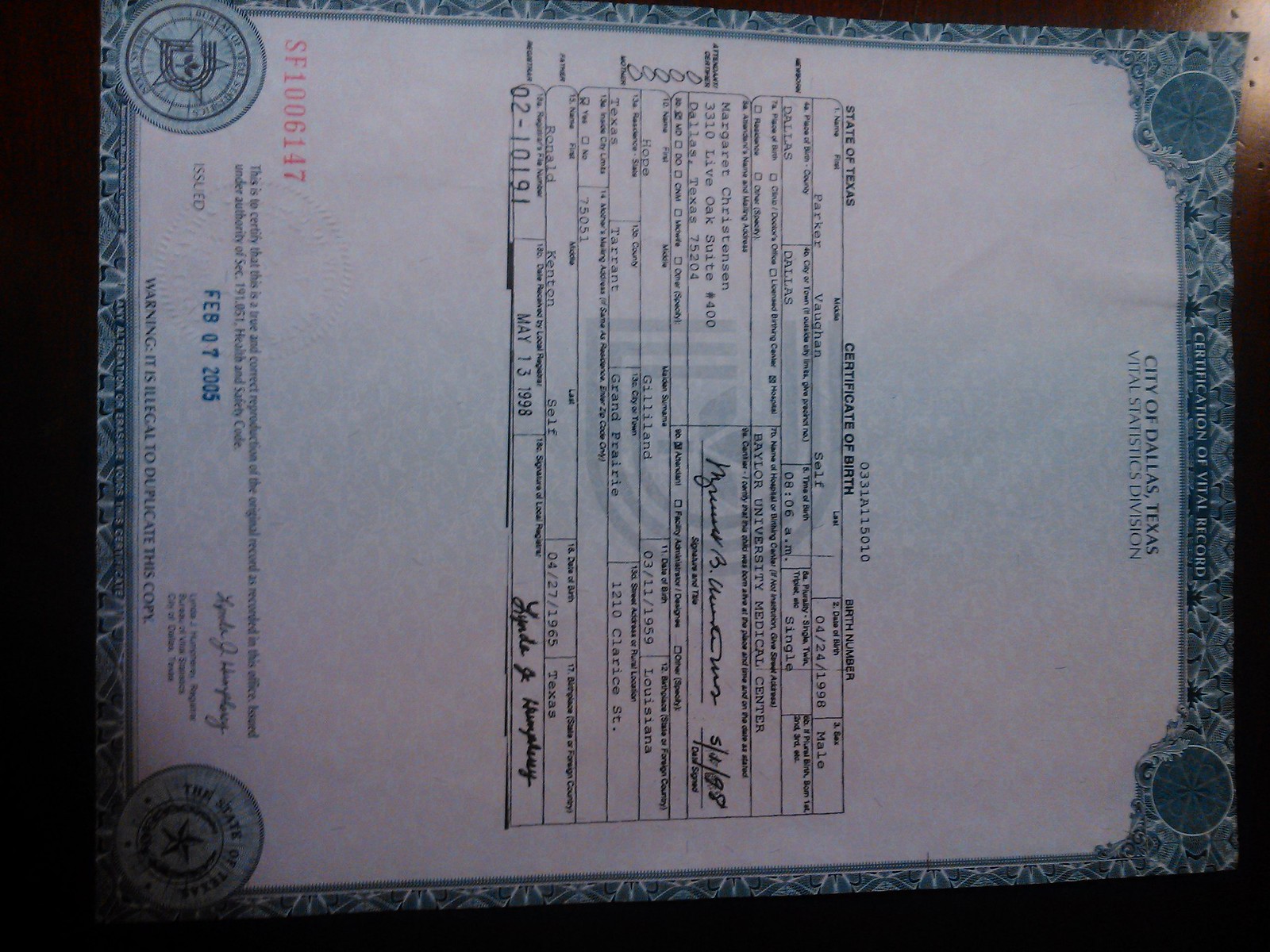The image is a detailed photograph of a birth certificate, positioned sideways and possibly lying flat on a brown surface. The document is predominantly white, featuring a noticeable blue border with decorative embroidery. At the top of the certificate, the words "Certification of Vital Record" are emblazoned in white, followed by "City of Dallas, Texas Vital Statistics Division" in black text. The form is titled "Certificate of Birth," and it includes various fields filled out with demographic information, including the name Seath Parker and the birth date of February 7th, 2005. Several boxes similar to those on an IRS form are thoroughly completed. At the bottom of the certificate, there are multiple dates, signatures, and a serial number in red. The overall colors in the image include brown, blue, white, black, and red, indicating the certificate's official and detailed appearance.